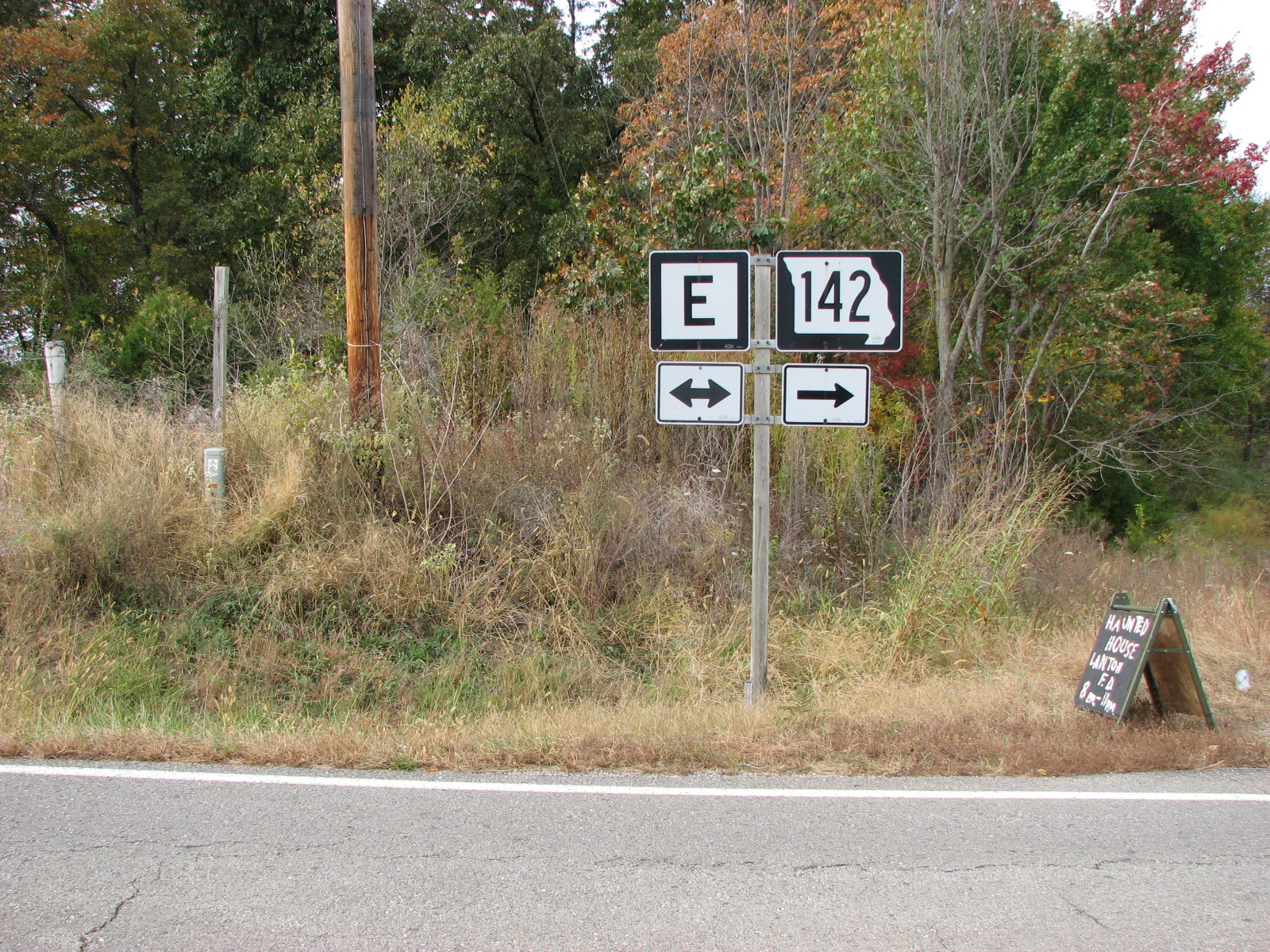The image depicts a roadside scene featuring a cracked pavement bordered by a white line that separates the road from a grassy field. Prominently positioned in the field is a multi-sign road post. At the top left, there's a white sign with a black border displaying the letter "E." Below this, another sign features a double-sided arrow. On the right, a sign illustrates the outline of a state with the number "142" in black text, accompanied by an arrow pointing right beneath it. The background comprises a wooded area with one leafless tree and others with full foliage, and a light pole can be seen to the left. Additionally, a small black sign, possibly advertising a haunted house, stands in the right corner of the image.